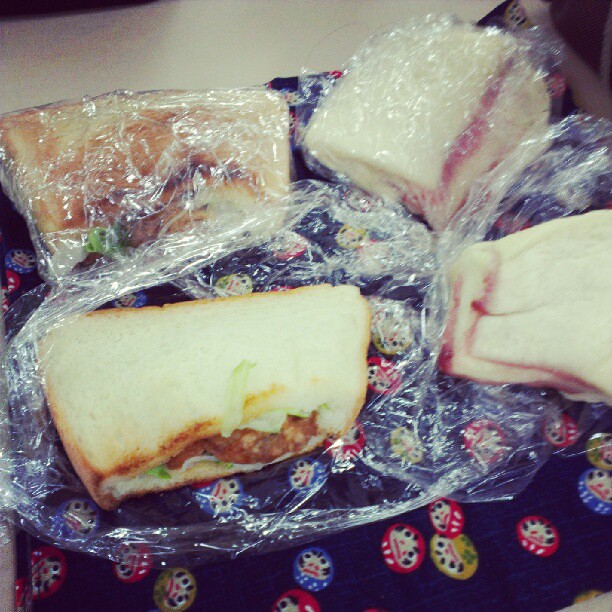This image depicts a scene at someone’s house, showcasing four sandwiches, three of which are wrapped in cling wrap, while one remains unwrapped at the forefront. The sandwiches are set on a dark blue plate adorned with whimsical, colorful prints that resemble small faces or animals. The designs feature a mix of blue, red, and yellow with white faces and black dots. The sandwiches themselves are made from notably white bread, possibly toasted, but their fillings are indiscernible, with one hinting at potentially containing bacon or lettuce. The background reveals a plain, white counter devoid of any additional elements or people, emphasizing the sandwiches as the focal point of the photograph.